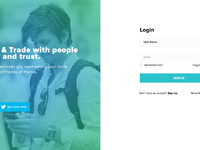The advertisement snippet appears on a mobile device screen against a greenish-blue background. Superimposed on this background is the image of a young man with somewhat long hair, looking down intently at his phone. He is dressed in a white shirt with sunglasses hanging from the collar and carries a backpack. 

The visual only captures the profile of the young man, highlighting one side of his head and body. In bold white print, the advertisement bears the phrase "Trade with people you trust," with an ampersand symbol replacing the word "and."

Further down, the layout includes a blue box whose details are difficult to discern. To the right, slightly darker print shows the word "Login" with a rectangle field intended for entering an ID, a password field, and a blue bar for signing in.